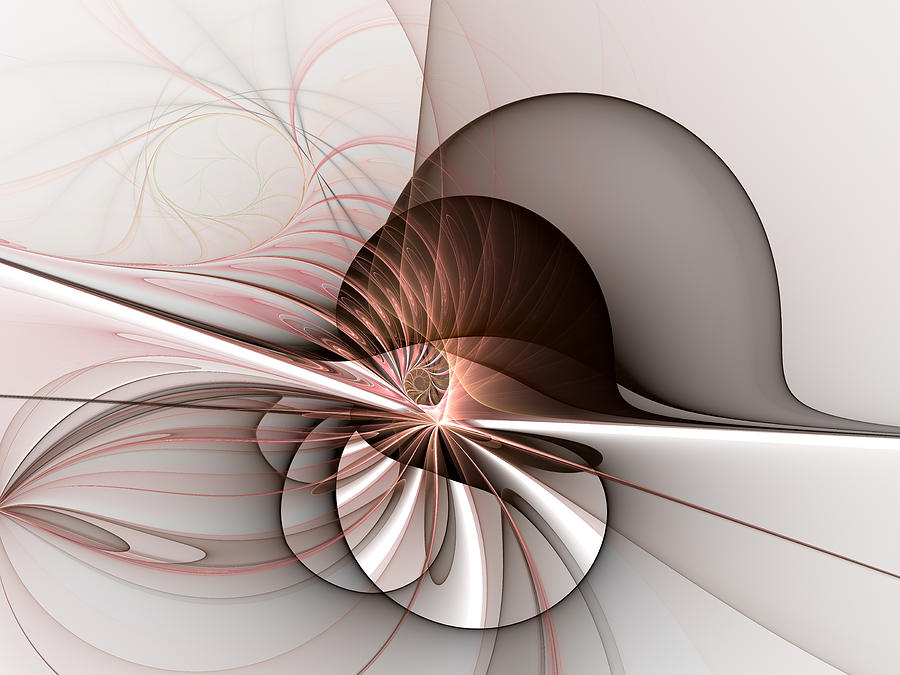The image is a highly detailed and intricate abstract painting, reminiscent of a seashell or snail shell rendered in a swirling, string-art style. The artwork features a predominant spiral structure at its center, evoking the natural geometry of a snail’s shell. Surrounding this central spiral are an array of smaller circular and oval shapes in varying shades of white, gray, and brown, creating a sense of movement and depth. The top left corner of the image showcases a primarily white background with delicate pink, reddish, and occasional orange streaks, adding a subtle warmth. As the eye moves to the right, the background transitions to beige, further enriched with a prominent gray half-circle that adds contrast and dimension. Below, the background darkens to gray, continuing the motif of swirling lines. Throughout the painting, diagonal brown lines intersect, enhancing the dynamic flow of the composition. The overall palette includes an earthy mix of browns, grays, whites, and beiges, punctuated with delicate hints of pink, blue, and orange, making this a striking and complex piece of abstract artwork.